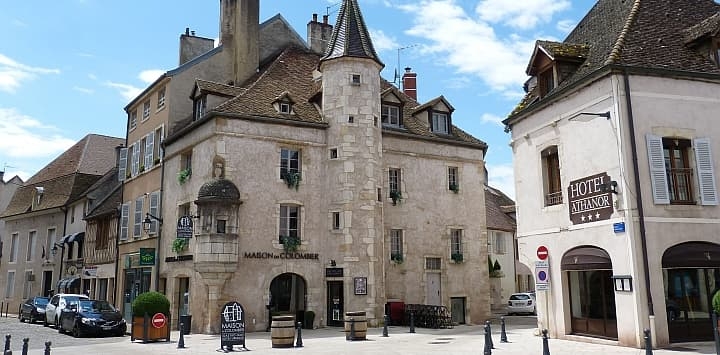The image showcases a charming street in a European city, potentially France, characterized by its older, stone-built architecture. Dominating the right side, a cream-colored building with a black, triangular roof and a brown sign that reads "Hotel Athenor" stands out. This building features large, beautiful windows with white shutters on the second floor, and entrances on both the left and right sides. Adjacent to this, towards the center and extending to the left, is a series of interconnected buildings, some resembling ancient castle-like structures typical of Greece or Italy, giving an impression of historic elegance. These buildings vary in color, predominantly beige and white, and differ in size. The street is cobbled with stone walkways and is dotted with parked cars on the bottom left and along an alley on the right side. Metal-wrapped barrels serve as trash cans, and several "Do Not Drive" and "Do Not Park" signs are visible. The sky above is light blue with a few scattered clouds, adding to the picturesque ambiance of this quaint European street.